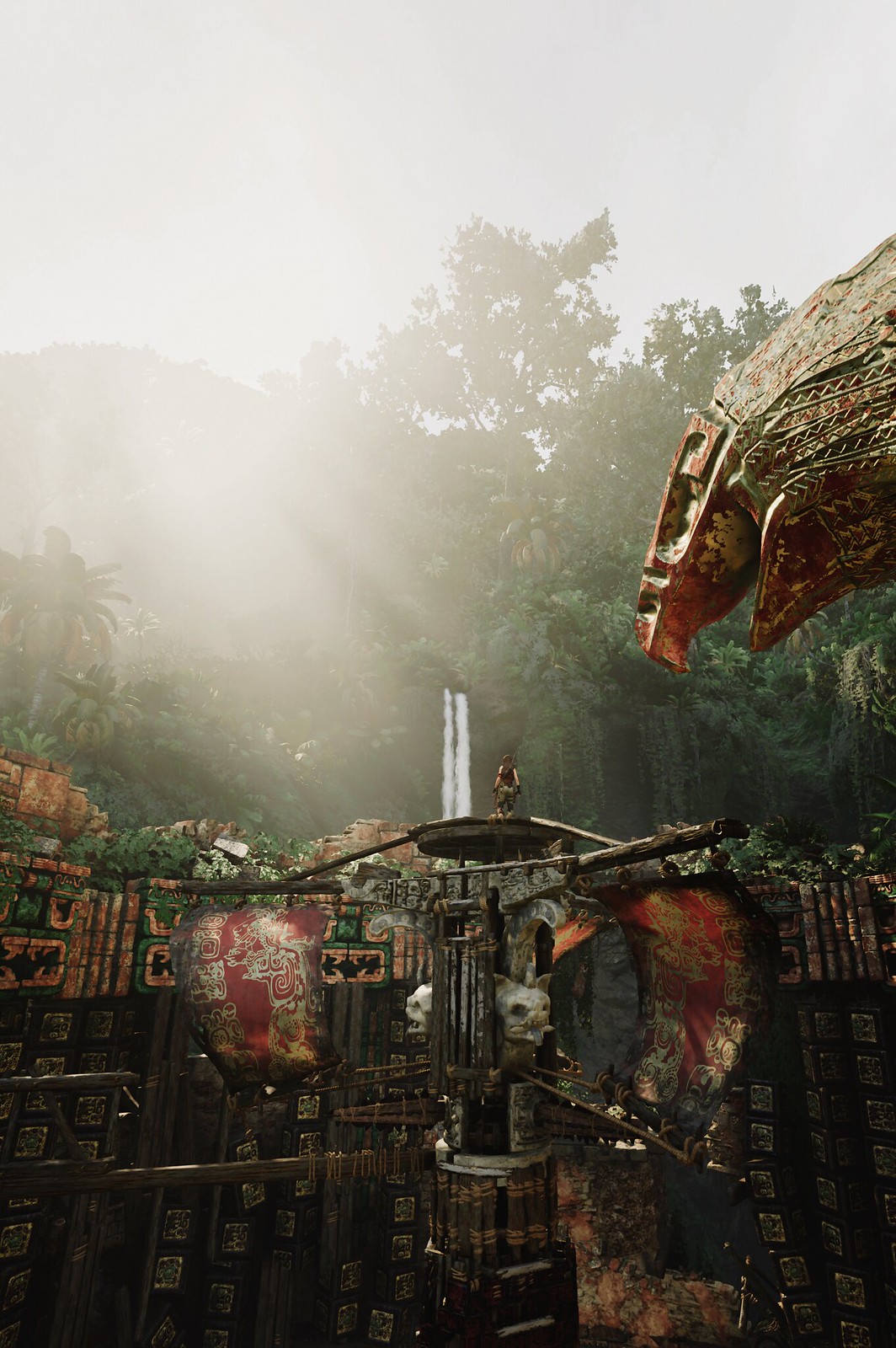The image presents a richly detailed scene that appears to straddle the line between an ancient and a fantastical setting. In the background, a cascading waterfall flows gracefully down through a lush, verdant forest, featuring both deciduous and tropical palm trees whose leaves bask in the bright sunlight breaking from the left side, creating a striking glare. The sky above is hazy, contributing to the scene's mystical ambiance.

Foreground elements introduce a man-made, fortress-like structure that exudes an ancient, perhaps re-imagined, architectural vibe. A notable feature is a circular lookout point where a human figure, clad in a black shirt and green pants, stands poised almost at the center of the image, aligning closely with the waterfall in the background. This lookout brings a sense of scale and interaction between human presence and the expansive, nature-filled surroundings.

Additionally, on the right side, a large, intricately designed eagle or falcon head emerges, cast in metal and soaring above the structures below. This bird motif continues with wrought iron fences adorned with skulls and books, adding to the otherworldly feel. Furthermore, there are flags and designs in gold and red that bring a pop of color and hint at cultural or symbolic significance.

All these details coalesce to create an enthralling tableau, reminiscent of a scene from a video game or a vivid imagination of an ancient urban legend, amplifying the visual narrative with its elaborate and cohesive elements.